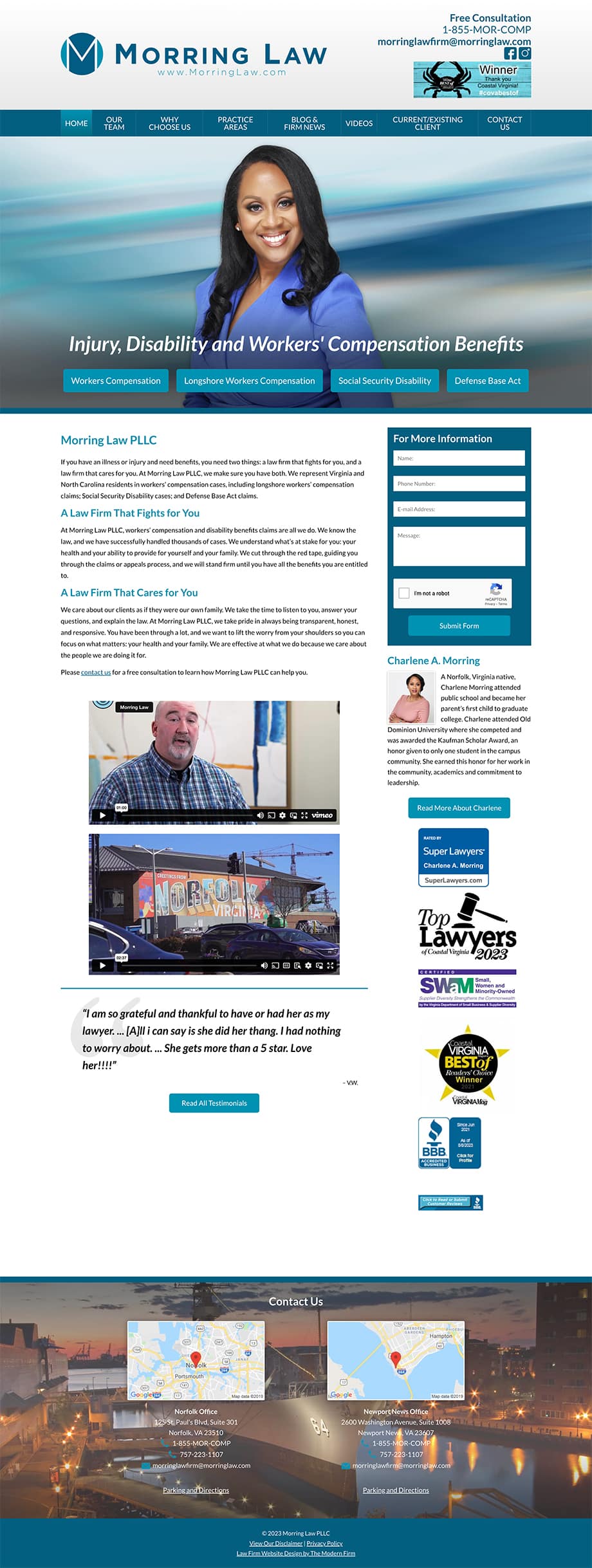The image showcases a law firm's website featuring "Morning Law" prominently at the top, with a distinctive "M" within a circle serving as the logo. Adjacent to this logo, there is the name of the law firm, accompanied by contact information, and an emblem resembling a crab placed within a blue rectangle that includes some text. 

Below these headings, there is a professional photograph of an African American woman, set against a softly blurred background that resembles an ocean scene. Beneath her image are the service areas listed: Injury, Disability, and Workers' Compensation Benefits. 

Above her photo, the site has navigation tabs leading to various sections of the website. Below her, there are three detailed paragraphs providing an overview of the website’s purpose and the services offered by the law firm. 

Next to these paragraphs, a contact form is provided for visitors to input their information and reach out to the firm. Following the descriptive text, the page features two video thumbnails. One video has a screenshot of a gentleman, while the other features a vehicle, offering visitors visual references and further information.

To the right of these videos are several recognitions and accolades, including Better Business Bureau Seals of Approval and Top Lawyer awards, though they appear slightly obscured. At the very bottom of the webpage, additional contact details and maps of the firm’s various locations are displayed, with an urban cityscape backdrop behind these elements.

This detailed arrangement and design suggest a professional, client-oriented approach aimed at providing easy access to critical information and services related to injury, disability, and workers' compensation benefits.